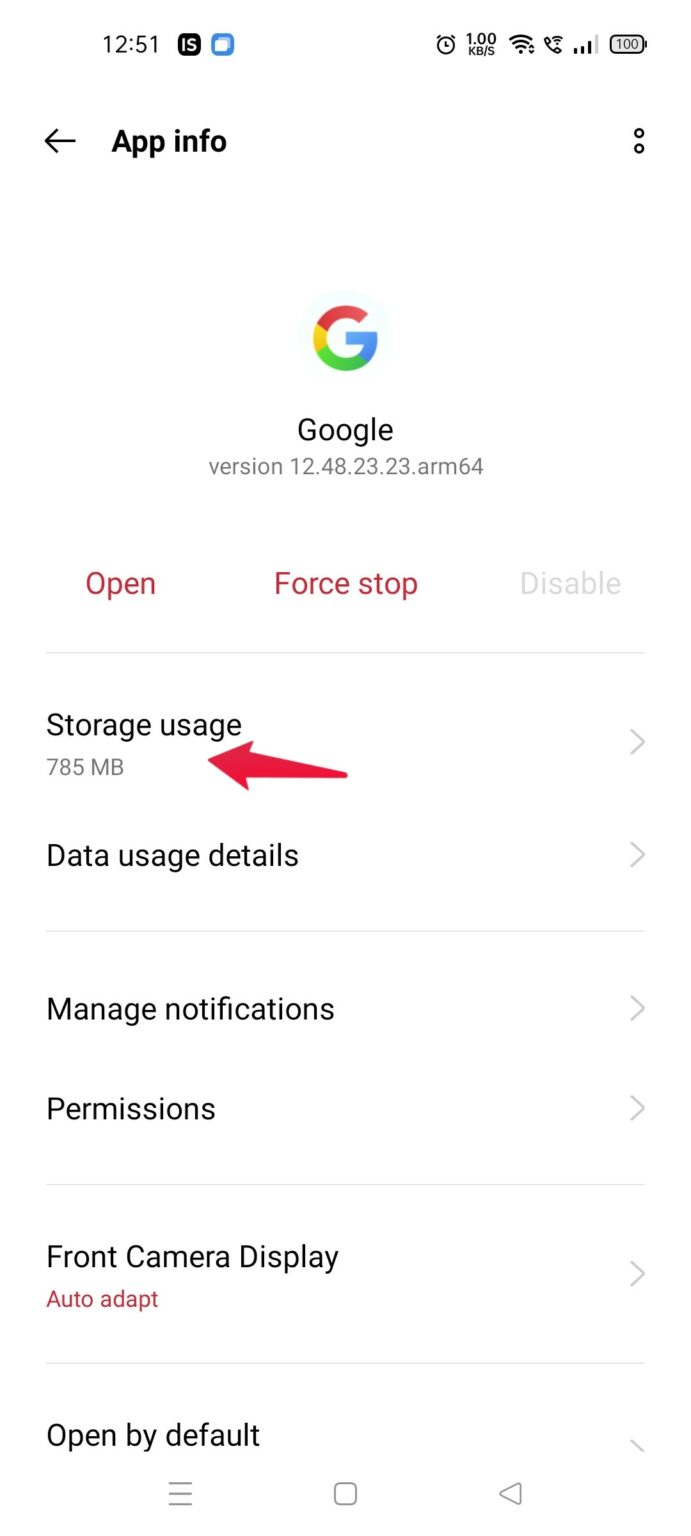This image is a screenshot of a cell phone, displaying the "App Info" page for the Google app on a white background. 

Top-left corner showcases the local time beside two small icons. The top-right corner features gray icons for phone functions: battery indicator, signal reception, and Wi-Fi status. 

Approximately three lines down and aligned left is a black arrow pointing left. Five spaces to its right, "App Info" is prominently displayed in bold black text. On the far right of this line, two thin, black-outlined circles are visible.

Centered four lines down, the Google logo (“G”) is displayed within a light blue circle, emblazoned with Google's colors. Directly below, "Google" appears in bold. Underneath, the text “version 12.48.23.23.ARM64” is presented in gray.

Three further lines down is a horizontally aligned menu with three options: a red "Open" on the left, a red "Force Stop" in the middle, and a gray "Disable" on the right. Below this menu, a light gray horizontal line separates sections.

The first section, labeled "Storage Usage" in bold black text, sits above the value “785MB” written in gray. A thick red arrow points leftward at the storage value, and a gray right-pointing arrow lies on the far right.

Next is "Data Usage Details" in bold black with an accompanying right arrow. Another horizontal light gray line separates this from the following section.

The next section titles in bold black are "Manage Notifications" and "Permissions," each paired with a right arrow.

A thin light gray line demarcates this from "Front Camera Display" in bold black text, with "Auto-Adapt" in red beneath it, followed by a right-facing arrow.

Finally, another gray line precedes "Open by Default" in bold black text, with the arrow partially visible to the right.